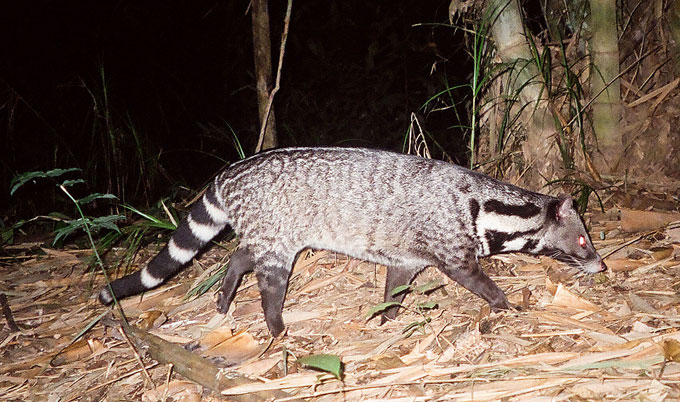In this nighttime photograph, a black and white civet is captured walking towards the right through a forest floor littered with brown leaves, bark, and plant debris. The animal's coat is a striking pattern of white and black, with its body mostly gray and splotchy, appearing almost striped at places, particularly around its neck and tail. Its legs are dark gray, and its eyes are glowing red-orange, likely reflecting the flash used by the wildlife photographer. The background is engulfed in darkness, indicative of the night sky, with various trees, including bamboo branches with green leaves, visible along the right side of the image. The ground shows a mix of dried leaves, twigs, and patches of brown dirt, framing this nocturnal scene in the dense forest.